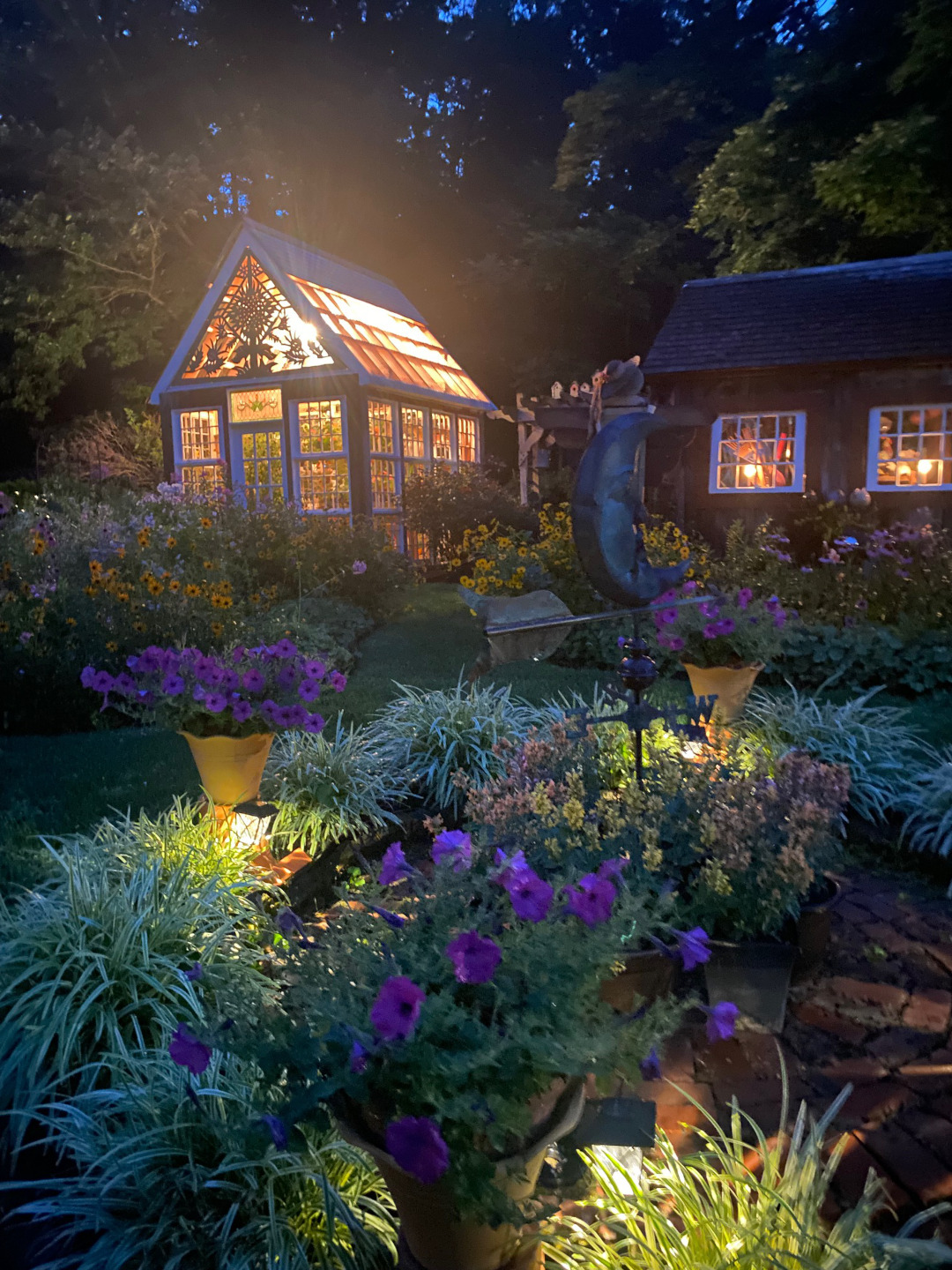The image captures a serene outdoor area of a house at night, showcasing a well-lit greenhouse on the left and the main house on the right. The main house features a sloping roof and white-framed windows glowing with a warm, orange light. The enchanting garden in the foreground is abundant with various plants and flowers, predominantly purple, with occasional patches of white, yellow, and orange blossoms. Garden lights cast an orange hue, enhancing the vibrancy of the greenery and flowers. Tall trees form a natural backdrop, and though it's a nighttime scene, a sliver of blue sky is faintly visible through the foliage. Brown rocks are interspersed among the plants, contributing to the overall rustic charm of the garden. The setting beautifully marries the elements of gardening and cozy outdoor ambiance.